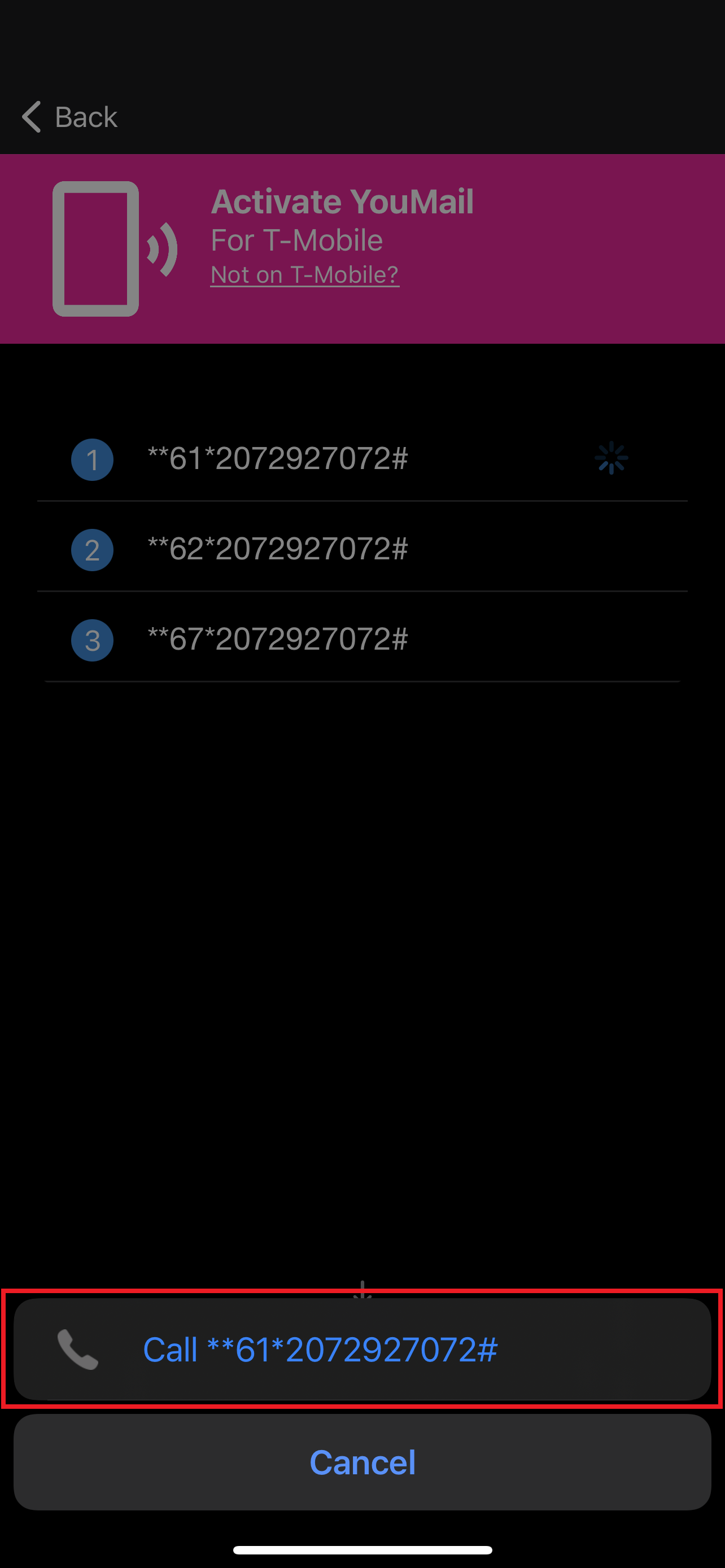This screenshot, captured from an older model iPhone, is evident from the use of sans-serif fonts and legacy interface elements. The image appears to be an edited screenshot intended for a tutorial. Dominating the lower portion of the screen are two prominent buttons. The first button, highlighted in red, reads "Call" and is followed by the code "**61*2072927072#". Below this, there is a "Cancel" button.

In the semi-transparent background, which appears greyed out, there are three instances of the same phone number, each labeled sequentially as 1, 2, and 3. The first number is selected, triggering the call menu overlay. Above this section and directly beneath a "Back" button, there is a pink banner that reads "Activate YouMail," with the letters 'Y' and 'M' capitalized. The banner specifies the service is "for T-Mobile." Below the T-Mobile message, there is a smaller, underlined link stating "Not on T-Mobile," intended for users on other networks to click.